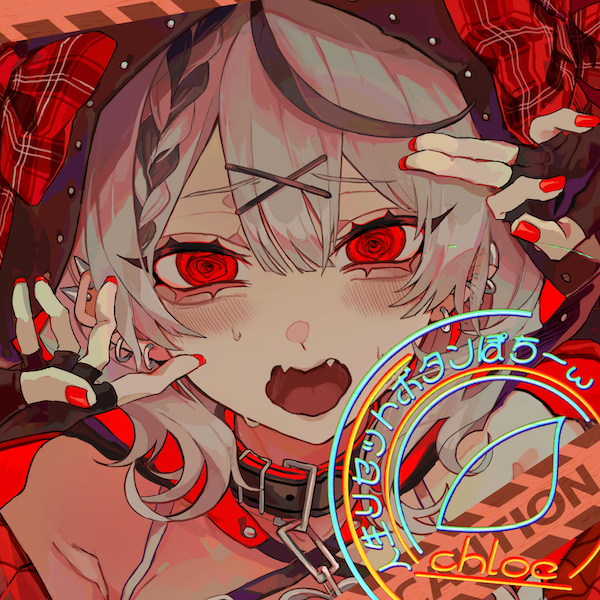This image is a digital screenshot of a haunting piece of artwork that portrays an anime-style depiction of an Asian female with gray hair, which partially features braids and plaid bows. The central figure has striking red, rose-like eyes and a light red nose. A prominent X mark is visible on the front of her bangs. She is depicted with a fierce expression, showing two sharp teeth on each side of her upper jaw. The person's attire includes fingerless gloves, red-painted nails, and a black and red collar connected by a chain, adding to the eerie ambiance. The overall color scheme is dominated by red and gray tones, creating a glowing, ominous atmosphere. In the bottom right corner, there is a captivating, neon-like inscription in Japanese, alongside the name Chloe written in glowing orange and red colors. The word "Caution" is also part of the text, heightening the sense of foreboding in the scene.